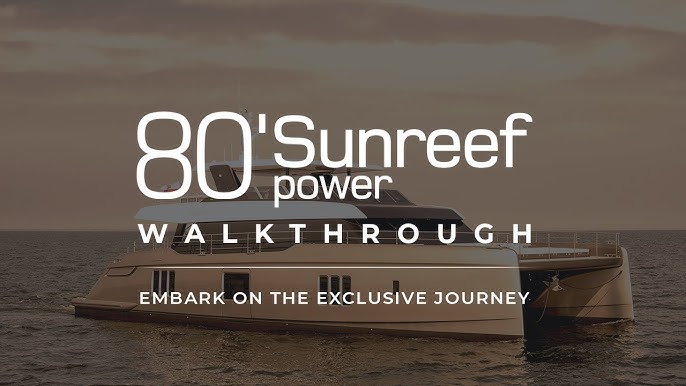The image is a dark, horizontal photograph featuring a large yacht or high-end watercraft situated on calm, expansive waters. Above, the sky is clouded, contributing to the image's subdued, dim ambiance. Dominating the scene are bold, superimposed texts in red and white that read: "80-Foot Sunreef Power." Below, in progressively smaller white letters, the phrases "Walkthrough" and "Embark on the Exclusive Journey" are prominently displayed, with a white line emphasizing 'Walkthrough.' The boat appears sleek and ultra-luxurious, with a rectangular, somewhat square shape and an indent suggesting an entryway or door. No birds, land, or people are visible, highlighting the vessel's solitude on the open sea under a cloudy sky, evoking an exclusive and serene journey.